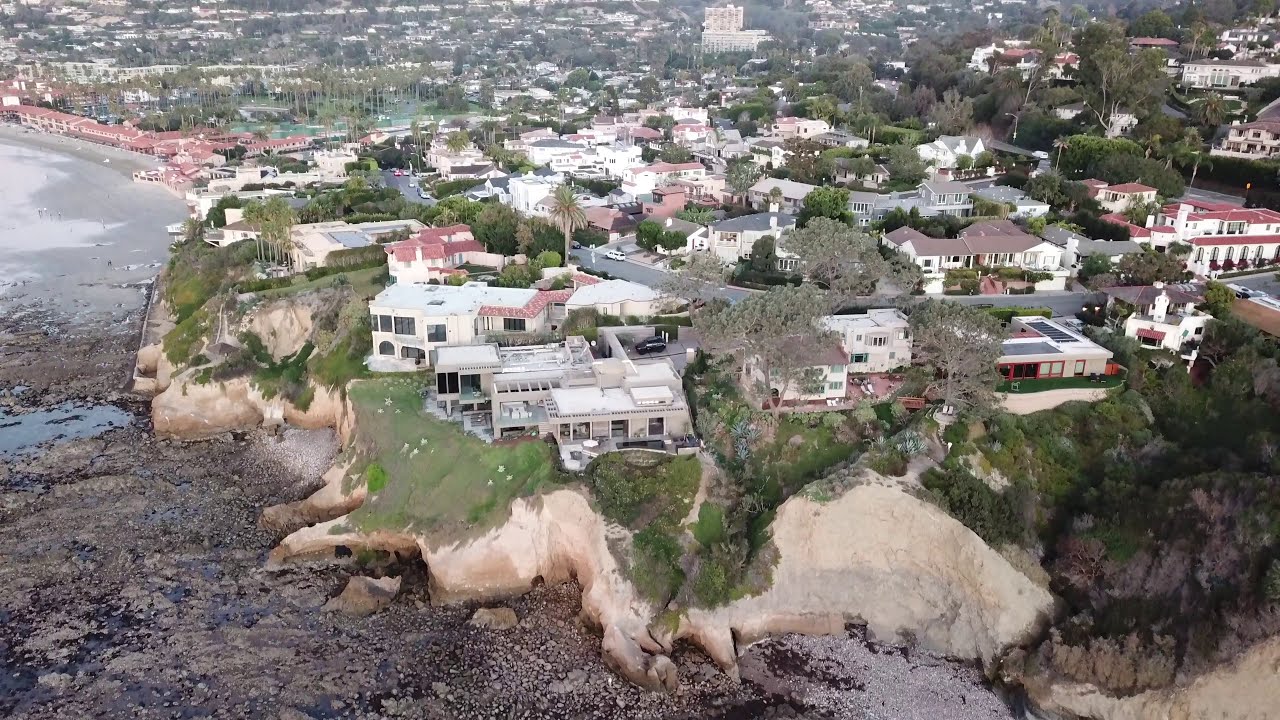This image is an aerial, overhead photograph of a distinctive, non-uniform community of two- and three-story houses. The houses are uniquely designed, varying in shape and style, and are situated on a rugged, craggy seaside landscape. In the foreground, houses are positioned on a large, grassy, and rocky jetty. To the left side of the image, there is a curved bay or seaside area, potentially an ocean or a bay, bordered by rocky land underneath high cliffs. The bodies of water appear potentially dried up, creating a landscape of gravel and mud rather than clear water. The community extends towards the right side of the image, with houses becoming smaller in the background, indicating more inland, landlocked areas. Despite no direct access to the water, all the houses are within walking distance to the bay area. The photograph captures the intricate layout and the unique positioning of the houses, highlighting the striking contrast between the rocky seaside and the closely built residential area.